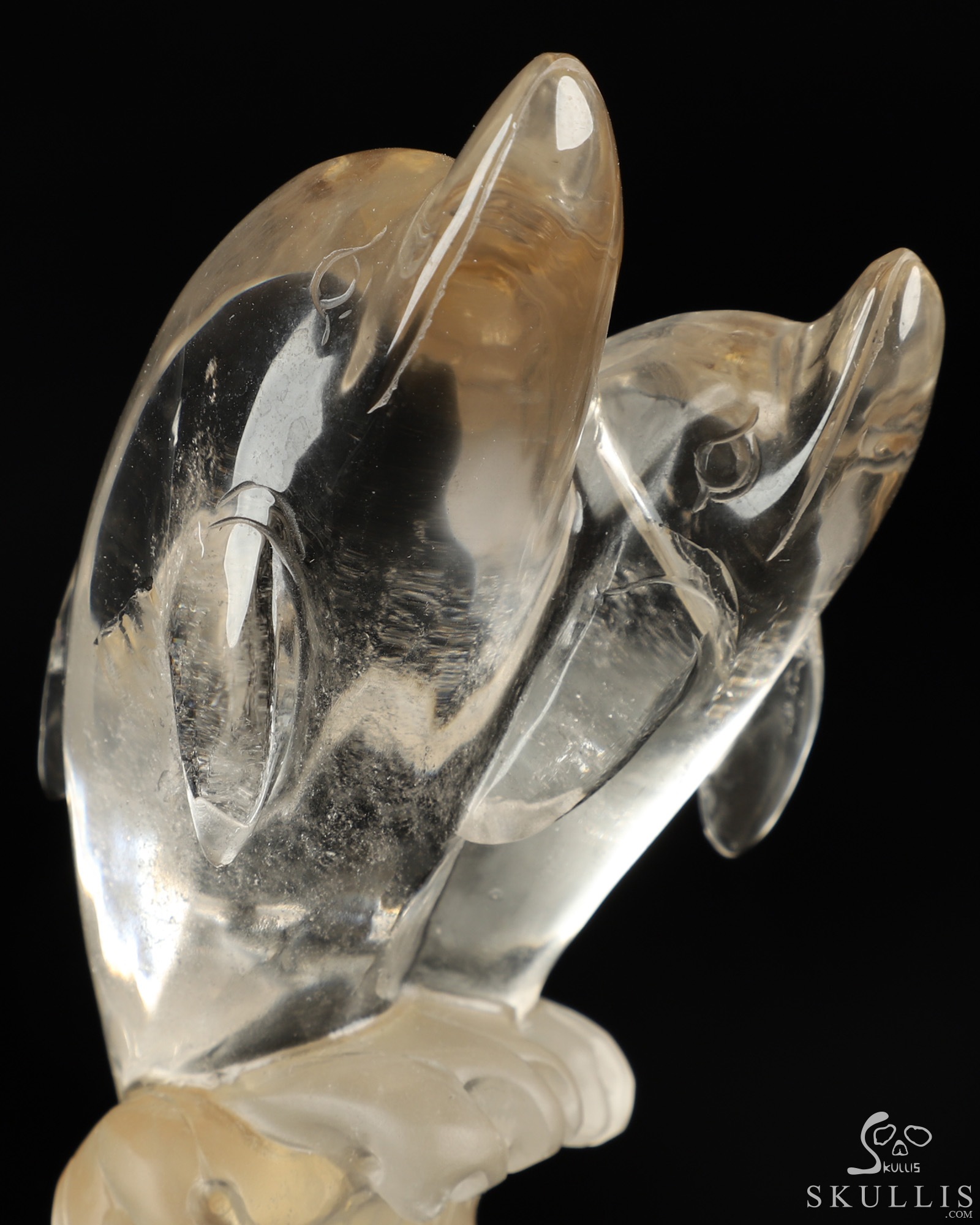The image showcases an impressive sculpture featuring two large, transparent dolphins. These dolphins, intricately crafted from what appears to be either ice or glass, exhibit a crystal-like, see-through quality, revealing details such as their eyes, noses, and fins. The dolphins, positioned as if emerging from a wave, rest atop a white base or podium, possibly held up by a hand, against a stark black background. Notably, on the bottom right of the image, there is a distinctive watermark displaying a small skull logo and the text "Skolas.com" in white, highlighting the artist's signature and website. The overall composition emphasizes the fine craftsmanship and clarity of the sculptures, making them both visually striking and exquisite.